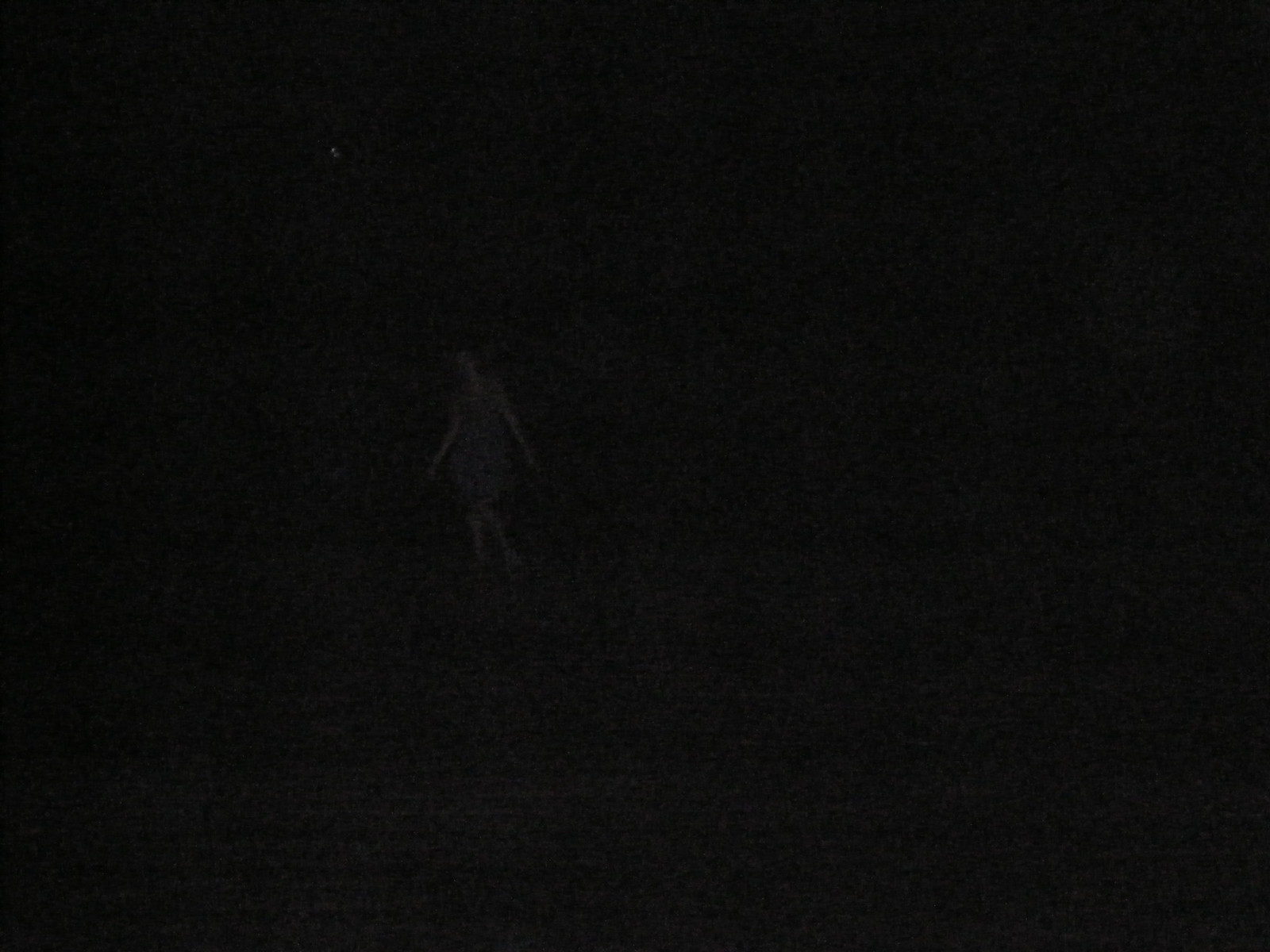In this photograph, the image predominantly features an almost pitch-black background with very dark grey shades interspersed throughout. The focal point is a faint, light grey outline of a person in the distance, seemingly a girl, possibly wearing a dress or shorts, with noticeably bare arms and legs visible from the knees down. Her arms are extended slightly out to her sides, and her head is subtly cocked to the left. The figure's knees appear to be slightly bent. Above her and to the left, there's a small, lighter dot, resembling a star in the night sky, which could either be an imperfection on the sheet or an intentional detail. The overall composition is minimalistic and shadowy, with the figure being the only discernible element against an otherwise dark expanse.